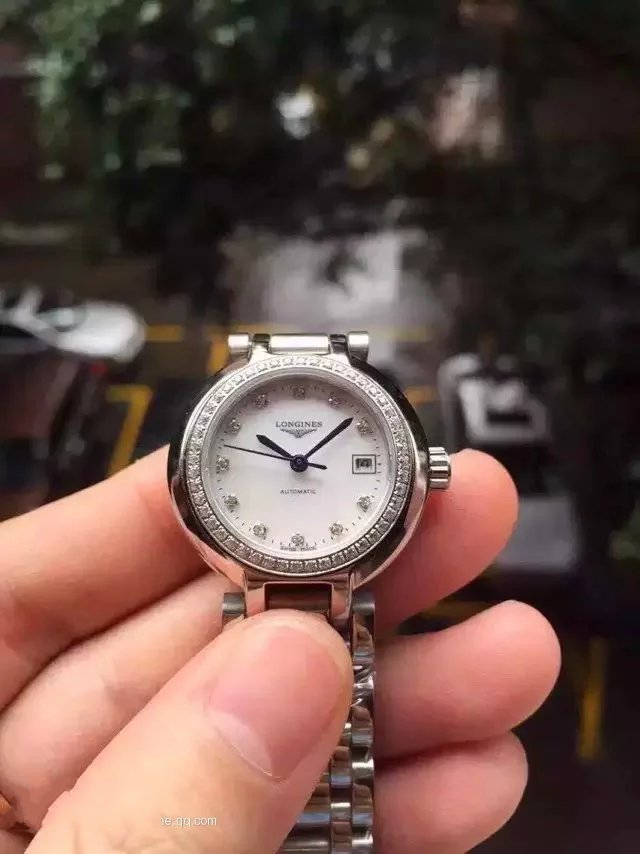In the photograph, a person's left hand with fair skin holds up an elegant luxury watch, prominently positioned toward the bottom left of the image. The watch features a metallic silver design with a chain-like pattern on its band. It boasts a rounded base with decorative rectangular patterns around its outer edge and a single silver knob to the right. The face of the watch is white and adorned with tiny silver crystals in place of numbers. There are three black, pointed hands indicating the time, which reads 10:09. The center of the watch includes the inscriptions "LONGINES" and "Automatic." The background reveals a scenic view of green trees and a parking lot with several cars, including a silver, a brown, and a white car, signifying that the image was likely taken from an elevated position. The thumb of the person holding the watch displays a partial text, "E.QQ.COM," in white.